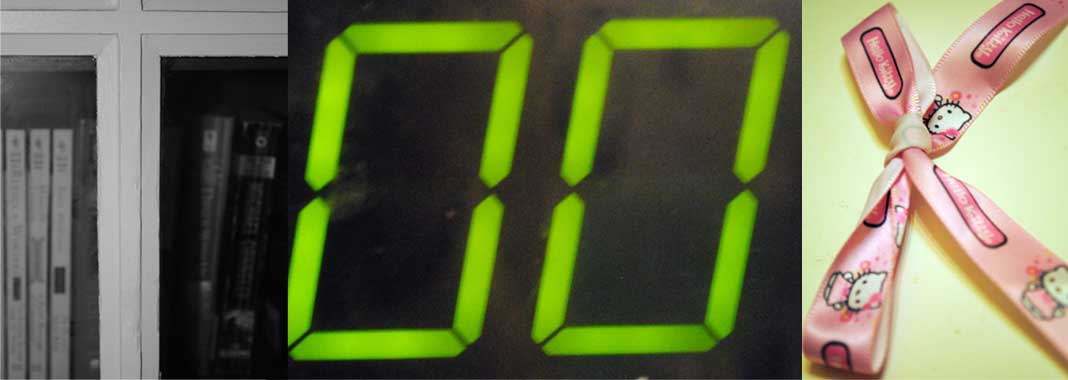The image is a wide, rectangular collage comprised of three distinct photographs, arranged from left to right. On the left side, the first photograph features a wall of a storage unit, revealing two separate cabinets. Within the left cabinet, three white books are neatly organized, while the right cabinet houses two thicker black books. The central section of the collage is a close-up shot of a green analog clock with a black background, where only the digits "00" are visible, likely indicating the seconds display. The rightmost photograph focuses on a Hello Kitty ribbon accessory. The ribbon is pink, adorned with the text "Hello Kitty" on each part and accompanied by an image of Hello Kitty in a pink dress with her iconic white cat head. The background of this right photograph is yellow, suggesting it might be resting on a table. The central image of the analog clock takes up approximately two-thirds of the total space, dominating the collage, while the left and right images each occupy about one-sixth of the area. This carefully composed collage juxtaposes elements of storage, time, and cute accessories, knit together in a visually intriguing arrangement.